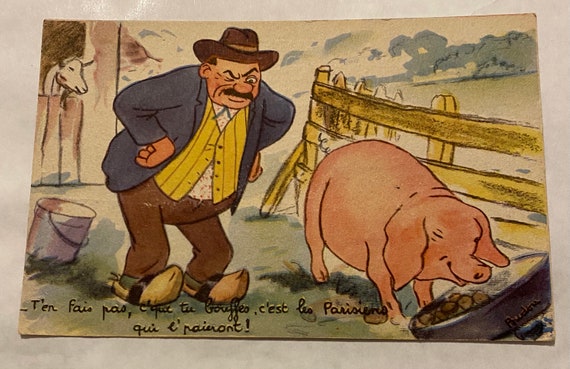This detailed cartoon drawing, resembling a watercolor illustration or a children’s storybook page, depicts a lively farm scene placed on a gray surface. At the center, there's a man dressed in a brown hat, dark blue jacket, yellow waistcoat, white shirt, brown pants, and yellow wooden shoes. He stands slightly crouched forward with his hands on his hips, one eye squinting and the other eyebrow raised, as he keenly observes a pink pig to his right.

The man, sporting a wide mustache, seems to have a bucket behind him and a goat peeking over a barn door positioned further in the background. The pig, with eyes closed, is eagerly eating food from a big black metal tray. A prominent yellow wooden fence runs to the right of the pig, supported by a beam on the left back end. Beyond the man and pig, the illustration captures a green farmland, lush with trees and hills forming a serene background.

Below the meticulous details of this scene, there is a small black French cursive text, slightly challenging to decipher but potentially important to the story being depicted.